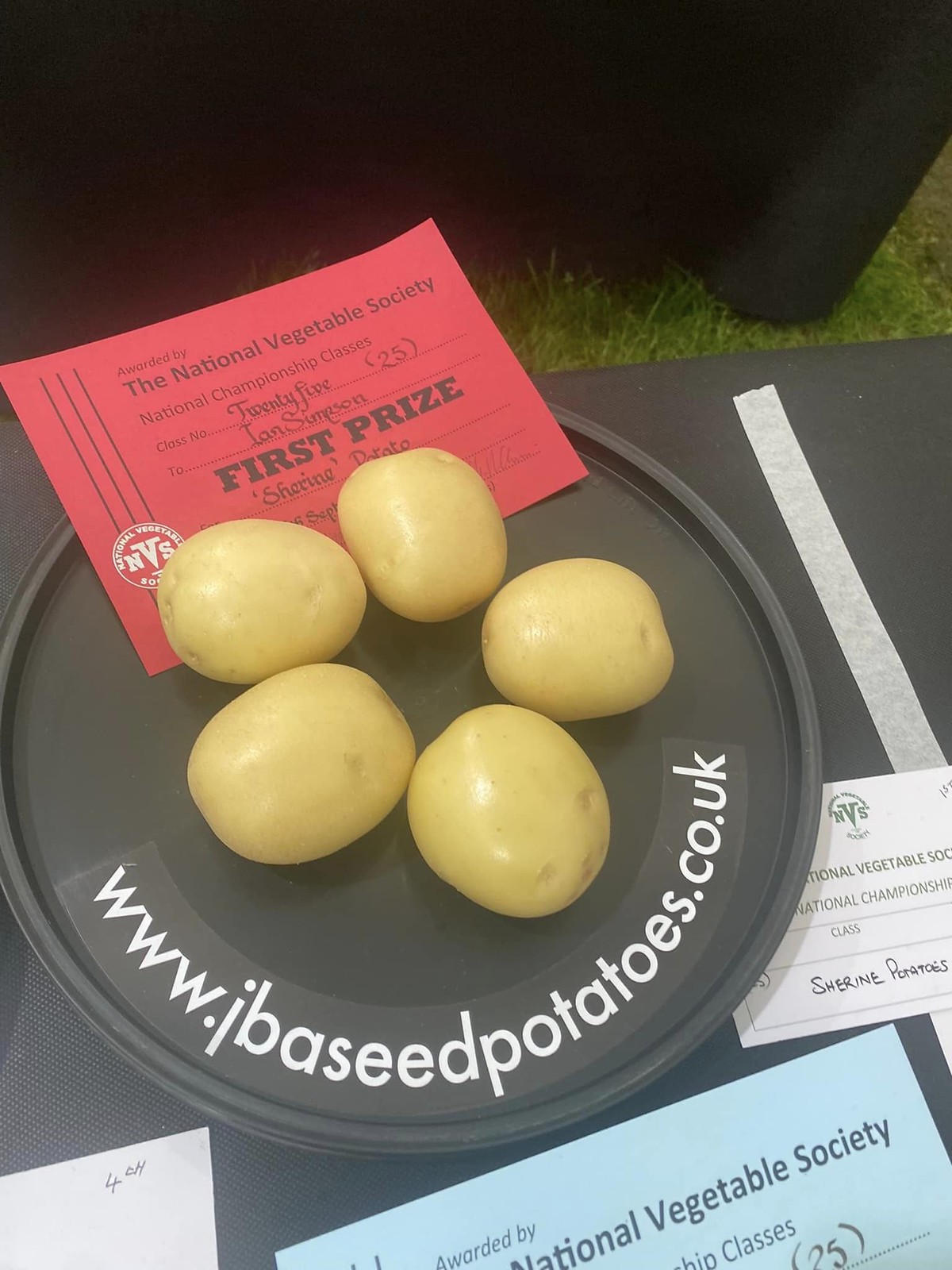The image showcases a photograph of a black circular platter displaying five smooth, golden potatoes arranged in a circle at its center. The platter features a red printed slip indicating it is an entry awarded by the National Vegetable Society under the National Championship Classes, specifically class number 25, where Ian Simpson secured first prize. Beneath the potatoes, the website "www.jbaseedpotatoes.co.uk" is visible. Additionally, at the bottom of the setup, there is a glimpse of another blue slip, likely pertaining to another entry in the vegetable competition.